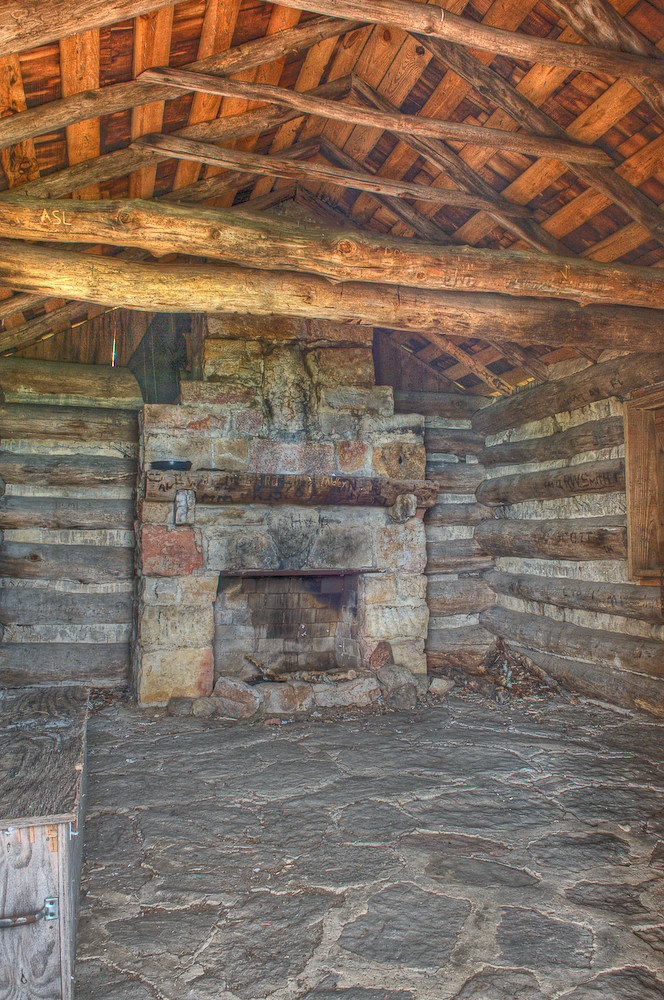This image is a detailed color photograph of the rustic interior of a log cabin, bathed in sunlight streaming from behind, likely through an open door. The floor is composed of irregularly shaped, gray flagstones meticulously fitted together with gray mortar. Dominating the far wall is a large, worn stone fireplace, constructed from a mixture of river-stone-like rocks and bricks, rising up seamlessly to form a chimney. Above it, a wooden mantelpiece, heavily etched with carved initials, stands prominently, exuding a sense of history and use.

The walls of the cabin are fashioned from long, split logs with flat sections filled in with wood or mortar, enhancing the authentic log cabin aesthetic. The high, pointed ceiling is supported by broad, hewn log beams, interspersed with wooden slats that showcase their grainy texture. Two massive logs act as crosspieces in the middle of the room, one of which bears the clearly carved letters "A-S-L."

On the left side of the room, there is a brown wooden table or bench, or possibly a box, made from weathered, old wood. This piece is distinctly functional, with a metal handle attached to its nearest end, reinforcing the room's rugged and utilitarian charm.